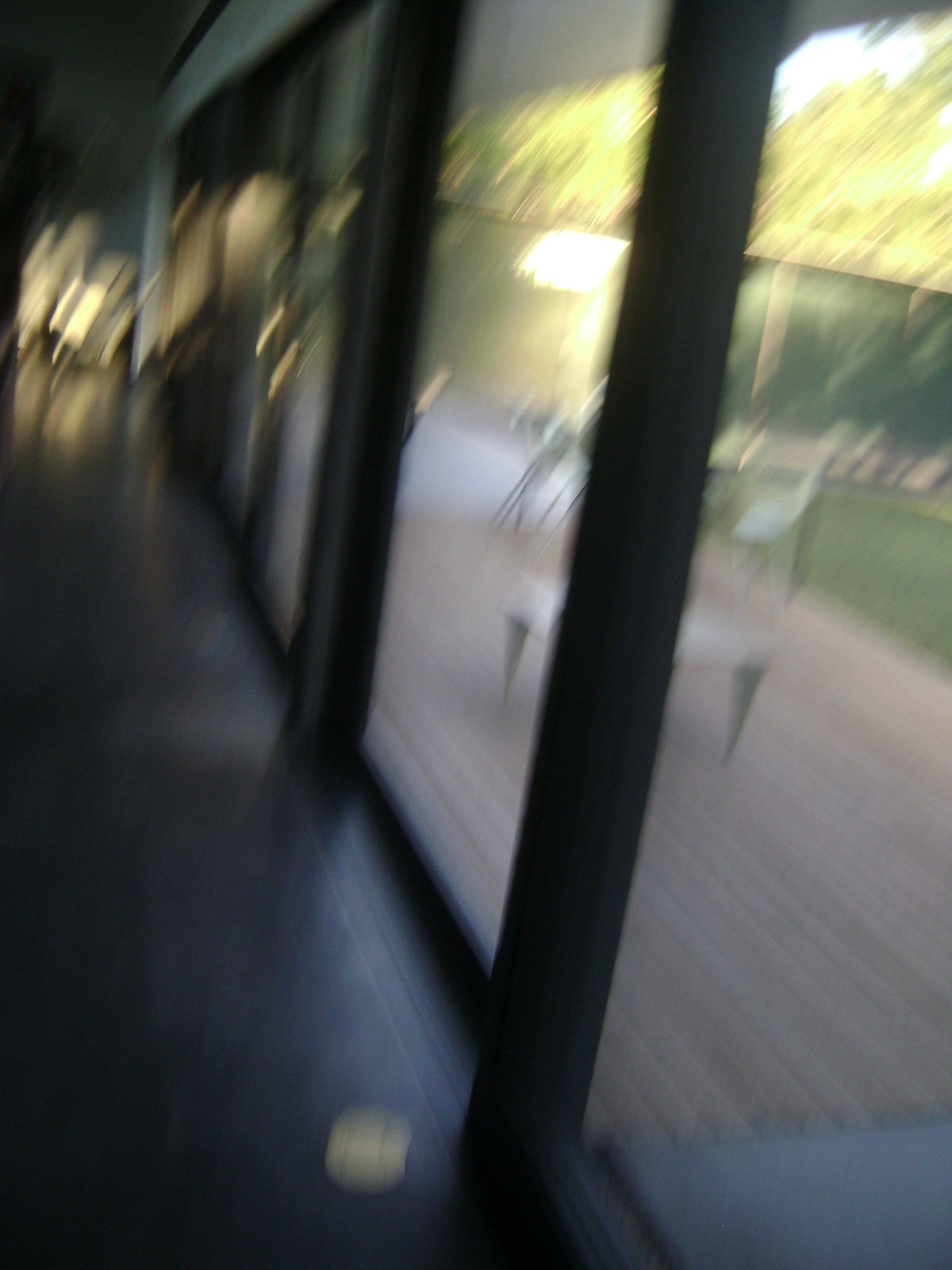This image depicts a partially indoor, partially outdoor scene viewed through a series of large, floor-to-ceiling windows along a hallway. The windows are framed by dark charcoal gray vertical pillars, creating sections of clear glass that blur the division between the interior and the exterior. The floor inside the hallway is made of dark gray tiles, possibly marble, enhancing the luxurious feel of the space. Outside the windows, there is a wooden deck constructed from thin strips of lighter brown wood. The deck features a round table with pin legs and several chairs positioned farther away, indicating a casual seating area. Beyond this outdoor deck, a privacy fence lines the background with trees full of bright green leaves peeking over the top and a sliver of pale blue sky visible above. There's also a small patch of darker green grass visible in the middle ground, contributing to the overall serene and inviting atmosphere of the setting despite the blurriness of the image.